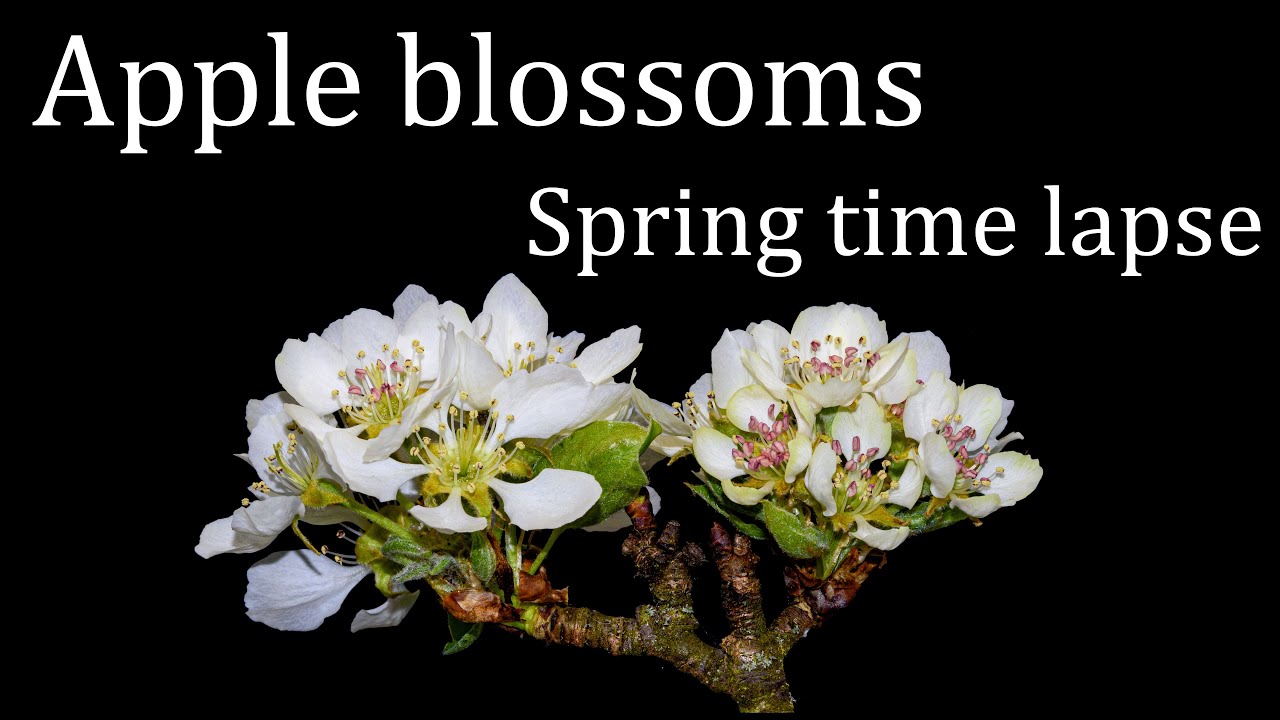The image features a stark black background with the words "Apple Blossoms" rendered in bold white letters at the top, and "Springtime Lapse" positioned slightly towards the right in the middle. Below the text, near the center of the image, a bonsai tree is depicted, adorned with small white flowers. These apple blossoms exhibit intricate details: the petals are primarily white with hints of green near the bottom, and the centers showcase pinkish to yellow hues. The blossoms are well-bloomed and are attached to brown branches, some of which have a dark grayish tone. Among the flowers, additional stems and roots extend visibly, contributing to the organic intricacy of the composition. The image is highly detailed and zooms in closely on the blossoms, offering a clear and vivid view of their structure and colors.